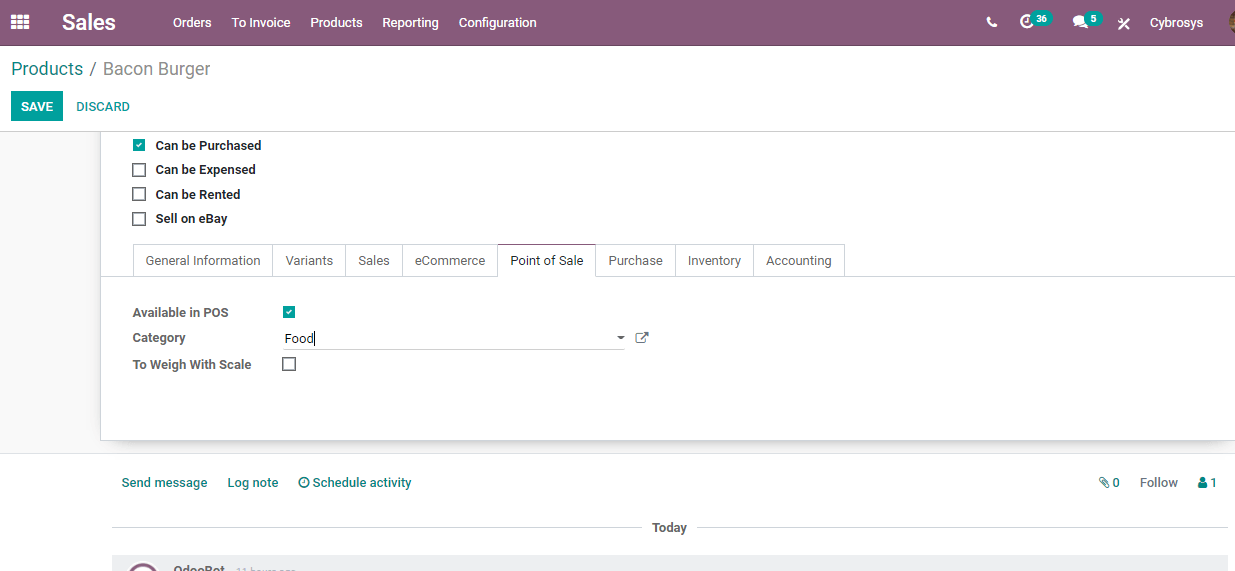The image displays a webpage with an organized layout, primarily in shades of deep rose and purplish hues. At the top, the header prominently features the word "Sales," followed by "Products," where "Bacon Burger" is specifically mentioned as an item available for purchase. 

Below the header, there are navigational tabs including "Orders," "Invoice," "Products," "Reporting," and "Configuration." In the upper right corner, there is a phone icon alongside a clock displaying the number 36 in green. Additionally, there are speech bubbles indicating that there are five messages awaiting review.

The page features a section titled "Cybro Sis," above a product section where the "Bacon Burger" is highlighted. Here, two green buttons offer options to either "Save" or "Discard." 

Further down, there are various checkboxes for additional product options. The "Can be purchased" box is checked, while options for "Can be expensed," "Can be rented," and "Sell on eBay" remain unchecked. The content continues with further descriptive text extending down the page.